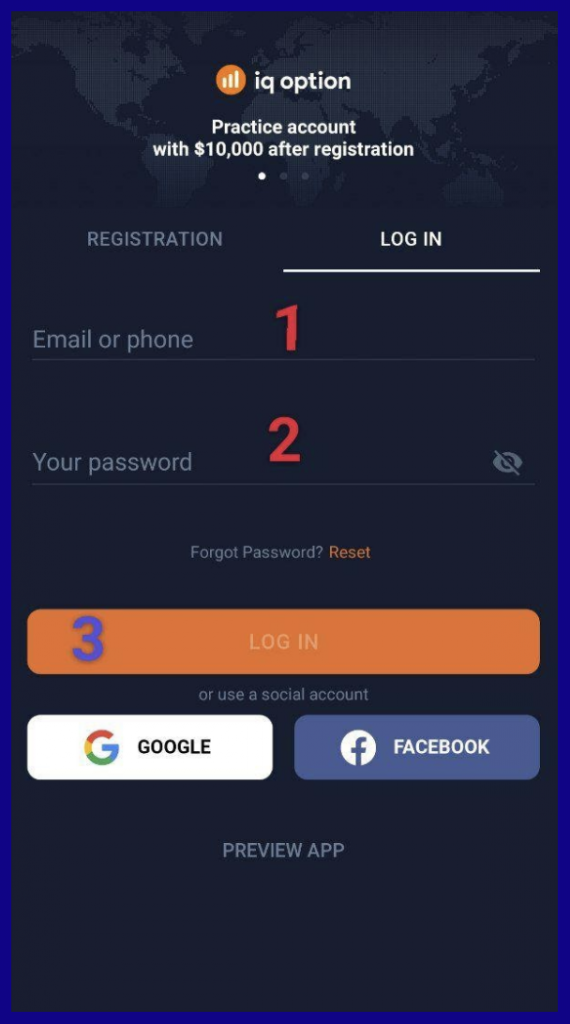Screenshot of the AppIQ mobile application login screen: 

The image depicts a login interface for the AppIQ application, with a practice account balance of $10,000 shown prominently following registration. The background is a navy blue shade, overlaying a faint world map graphic in gray behind the app’s name and the account balance indicator. 

Instructions for logging in are clearly numbered: 
1. Users can enter their e-mail address or phone number in the first input field.
2. The password entry field appears as the second step.
3. The third step involves clicking the bright and colorful login button.

Additionally, alternative login options are available at the bottom of the screen, featuring buttons for signing in via Google or Facebook, highlighted with their respective colors. However, the screenshot emphasizes using the traditional method of e-mail and password for this login tutorial.